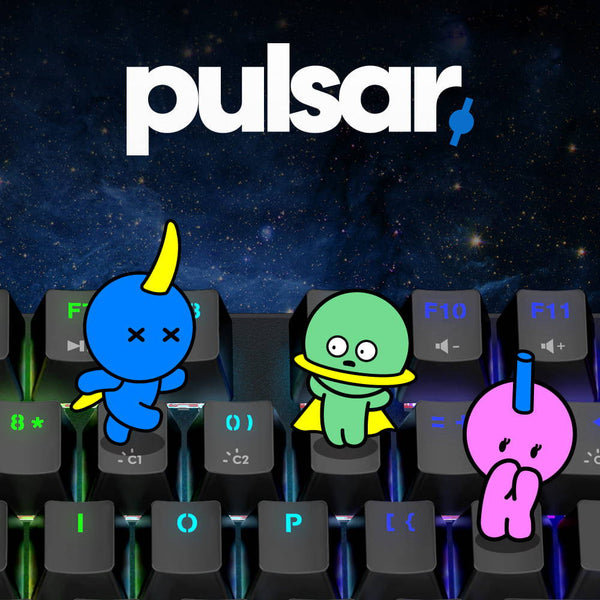The image, which appears to be an advertisement for a video game or cartoon, features prominently positioned text at the top that reads "Pulsar" in large white letters. Just to the lower right of this text, a small, medium-blue object resembling an ab roller is slightly tilted to the right. Behind this, a captivating space scene transitions from a dark blue in the upper right to a light blue in the lower left, indicating that the light source is emanating from the bottom left. The starry background contains peachy-colored stars that enhance the otherworldly atmosphere.

Occupying the lower half of the image is a zoomed-in section of a keyboard featuring approximately five or six keys in three rows. The keys are vividly colored, ranging from green to teal to a dark purple-blue. On top of these keys, three animated characters with cartoonish features are depicted. The character on the left is blue with a yellow cape, a horn, and appears to have two eyes. The middle character is green with a ring around the middle of its head and also wears a yellow cape. The character on the right is pinkish-purple, featuring a blue cylindrical object on its head and bashfully covering its mouth with its hands.

The vibrant and animated elements create a playful yet intriguing contrast with the vast, dark expanse of space in the background, drawing viewers into the fantastical world of "Pulsar."